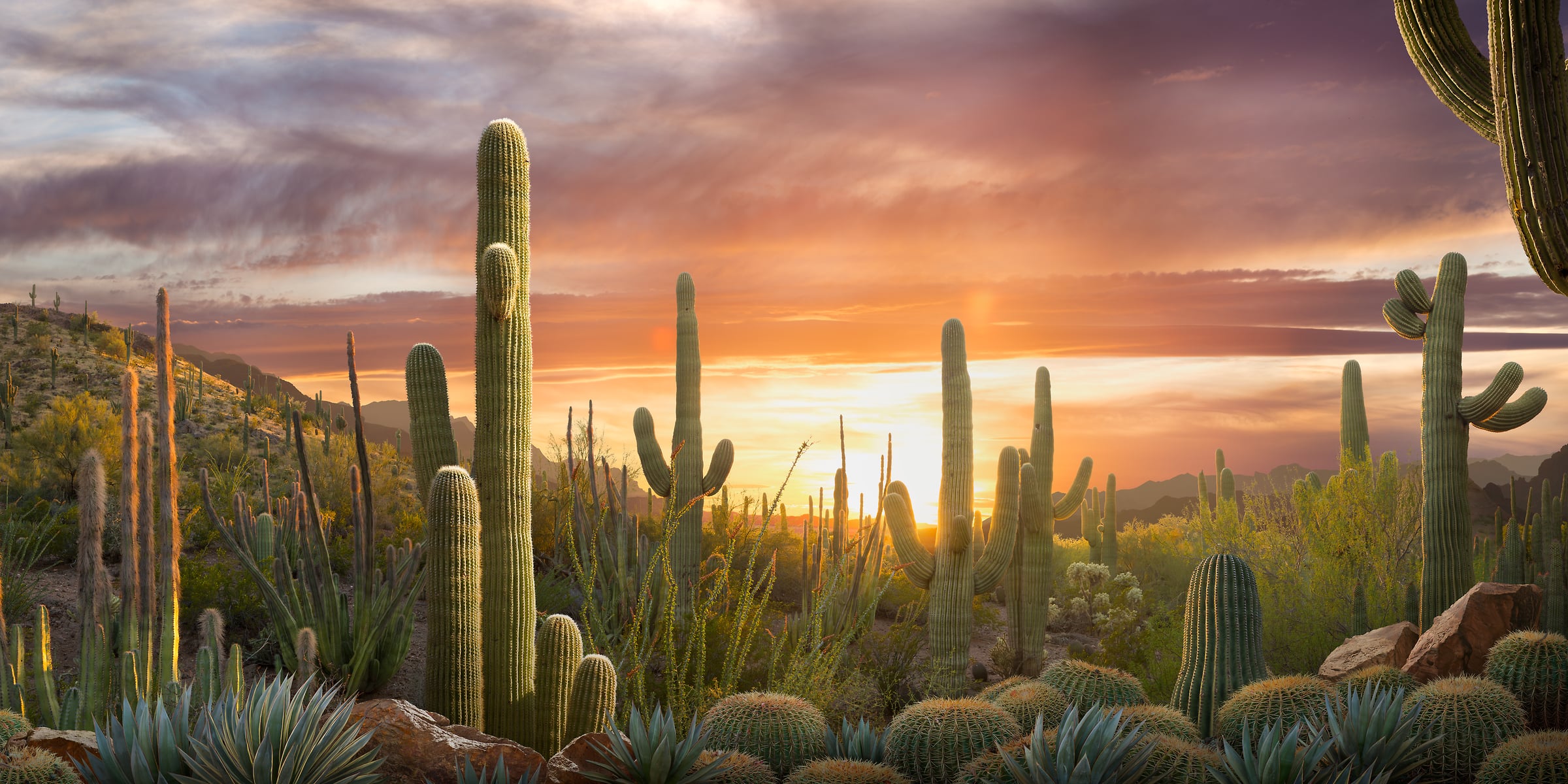This detailed depiction showcases a beautifully rendered desert landscape at sunset, brimming with diverse cacti and desert flora. The sky radiates a gradient of rich hues, shifting from a deep amber at the horizon to shades of purple and soft blue through scattered clouds. In the foreground, a variety of cacti are prominently featured, including tall, thin cacti about four to five feet in height, some with offshoots, and shorter, rounder cacti covered in spiky bristles. Interspersed among them are several aloe-like plants with stick-like leaves. The landscape is dotted with medium-sized red rocks and speckled with shrubs. Additionally, some cacti bear purple flowers, adding a burst of color to the verdant desert scene. The overall ambience is one of serene beauty, as the setting sun casts a warm glow over the entire vista, blending the reds, oranges, and purples in the sky into a breathtaking tableau, framed by distant hills.